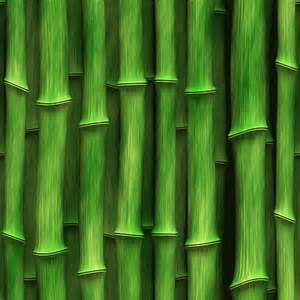This square-shaped indoor color image showcases approximately seven to eight vertical stalks of bamboo in a close-up layout. The bamboo is densely packed, filling the entire frame and creating an almost alternating row effect. Each stalk displays the characteristic bamboo ridging spaced at regular intervals, forming nearly two horizontal rows. The primary color palette is light green with pale green segments, highlighted by dark green shading in the background. The bamboo boasts slight striations and vertical striping patterns, with light tannin streaks and occasional spots of black shading between the stalks. This gives the bamboo an almost digital or painted impression. The image presents the bamboo in a natural state, with the stalks extending from the top to the bottom out of the frame, capturing intricate details such as the segment ridges and color variations. No text or print is present in the image.